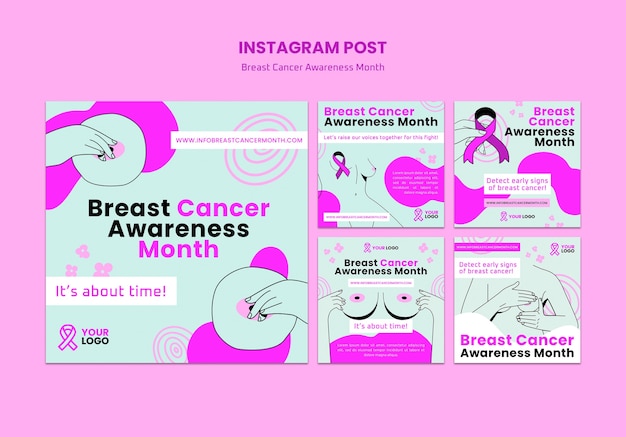The image features a prominent pink rectangle with bold purple text at the top reading "Instagram Post" and "Breast Cancer Awareness Month" underneath it. On the left-hand side of the pink rectangle, there is a large light blue box containing several elements. This box includes the text "Breast Cancer Awareness Month," alongside the phrases "It's About Time" and "Your Logo." Within this box, a pair of cartoon fingers appears to be performing a breast self-exam. Also in the top right corner of the blue box is the website address "www.infobreastcancermonth.com."

To the right of this sizable blue box are four smaller blue boxes aligned vertically within the pink rectangle. Each smaller box carries a distinct but related message:

1. The first small blue box states: "Breast Cancer Awareness Month. Let's raise our voices together for this fight." Some text and a website, rendered too blurry to read, follow this message.
2. The second small blue box reads: "Breast Cancer Awareness Month. Detect early signs of breast cancer," accompanied by additional, unreadable text.
3. The third small blue box repeats "Breast Cancer Awareness Month," shows cartoon hands performing a self-exam on a pair of breasts, includes the phrase "It's About Time," and has further, blurry text at the bottom.
4. The fourth and final small blue box contains: "Detect early signs of breast cancer. Breast Cancer Awareness Month," featuring a cartoon representation of a woman performing a breast self-exam.

Overall, the image uses a combination of clear messages and illustrative cartoons to emphasize the importance of breast cancer awareness and early detection.